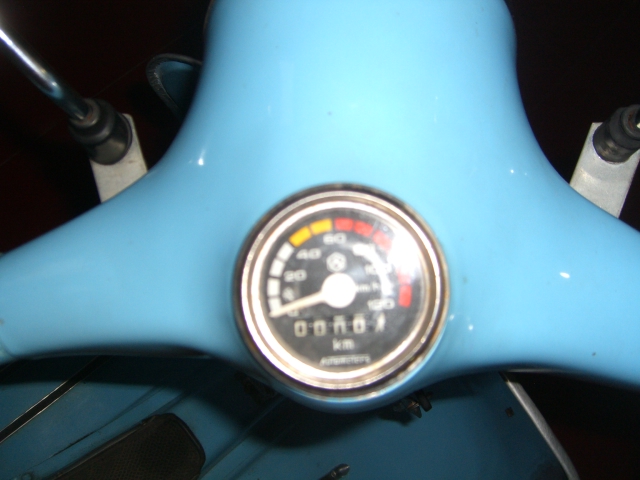An aerial photograph captures a mechanical instrument, prominently featuring a circular gauge mounted on an aqua-colored apparatus, which could be constructed of either metal or plastic. The gauge indicates measurement in kilometers, extending from 0 to 120 kilometers. Despite a slight blur, the gauge’s color-coded sections are discernible: 0 to 40 kilometers in white, 40 to 60 kilometers in yellow, and 60 to 120 kilometers in red. The gauge’s white dial suggests minimal usage, likely just beginning its first kilometer. The aqua-colored instrument rests upon another blue object, possibly a bag, distinguished by a visible black mesh component. Additionally, two white metal pieces with bolts at their bases extend upward from beneath the aqua apparatus, providing structural support.